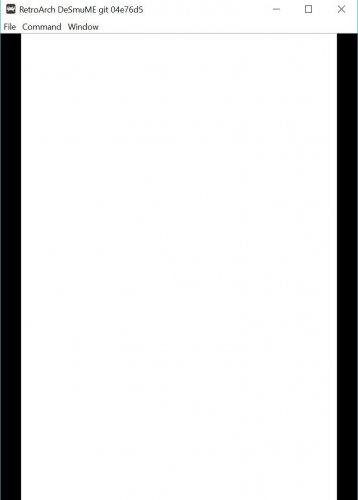The image is a blank white screenshot that appears to be a tall rectangle, resembling the dimensions of a mobile device. However, it could also be a screenshot of an app window with similar proportions on a desktop. On either side of the main content area are thick black bars running vertically down the left and right sides. 

At the top of the image, there is a header featuring a white background with black text. In the upper-left corner of the header, there is a black logo depicting a video game character made out of white pixels. To the right of this logo, the text reads "Retroarch DESMUME GET 04E76 DS." The text "Retroarch" is one word, and "DESMUME" is stylized with the letters 'S,' 'M,' and 'E' capitalized. Following this, the text "GET 04E76 DS" is displayed.

On the right-hand side of the header, the standard window control icons are visible: the minimize icon, the maximize icon, and the 'X' icon to close the window.

Below the header, there are three tabs labeled "File," "Command," and "Window," each with drop-down menus. The main body of the image beneath these tabs is entirely white space, with no additional content or details.